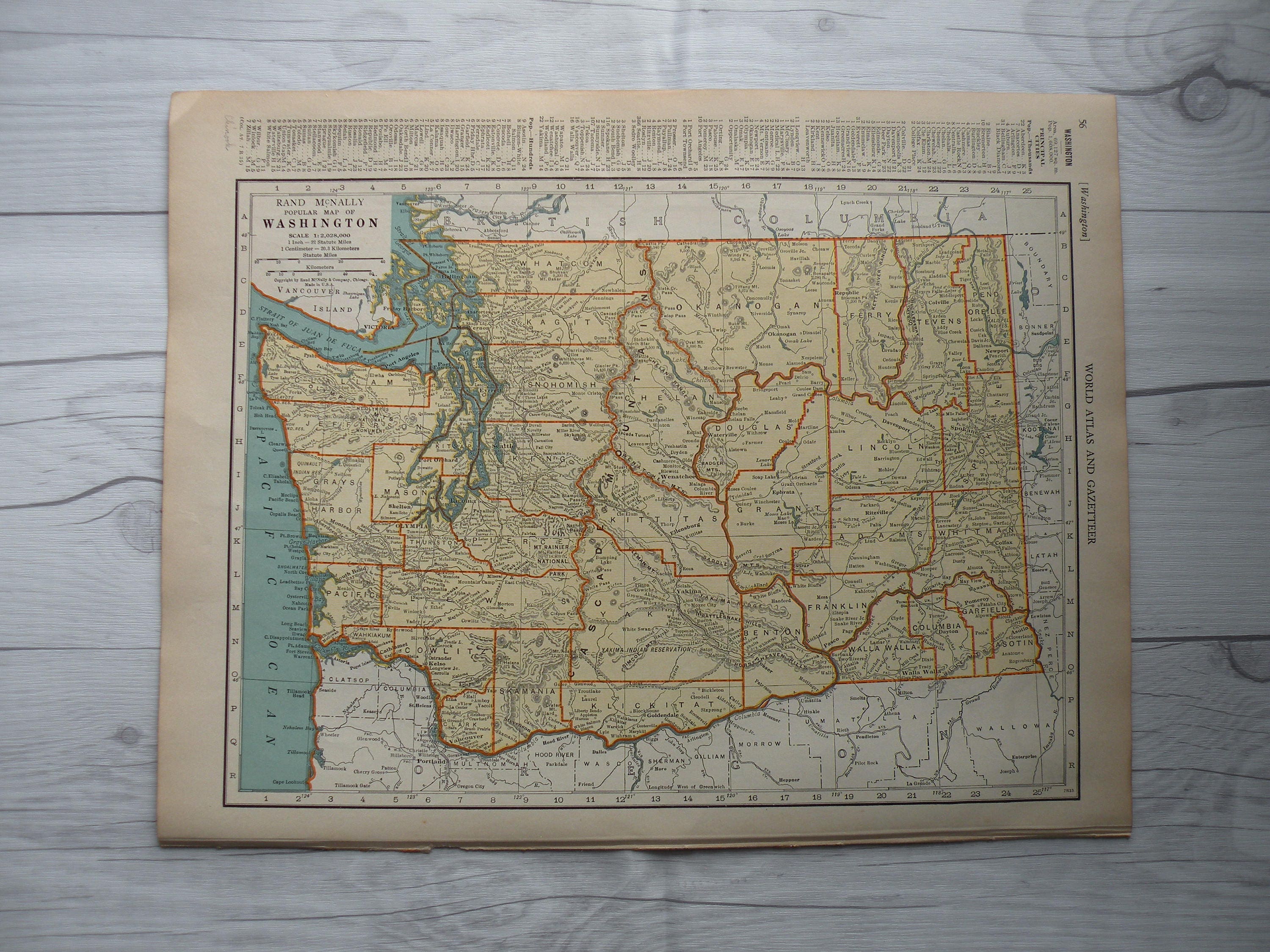This image displays a detailed map of the state of Washington, taken from a Rand McNally Atlas, positioned in a landscape orientation. The map, a wide vertical rectangle, is presented on a gray wood plank background, resembling either a floor or a wall. The main map is printed on a light brown piece of paper, outlined by a smaller black-trimmed rectangle.

Within this black rectangle, the state of Washington is prominently featured. It is outlined in dark orange and filled with a pale yellow color. The map is subdivided into various counties, all clearly labeled. Surrounding the state, the regions are depicted in white, with the ocean on the left side illustrated in teal blue.

At the top left-hand corner of the map, "Rand McNally Popular Map of Washington" and scale information are printed. Above this, a tiny, difficult-to-read key provides additional details about the cities and locations marked on the map. The top part of the map also includes text referring to a "World Atlas and Gazette." This detailed depiction encapsulates geographical and cartographical highlights of Washington State, complete with labeled towns and surrounding features.